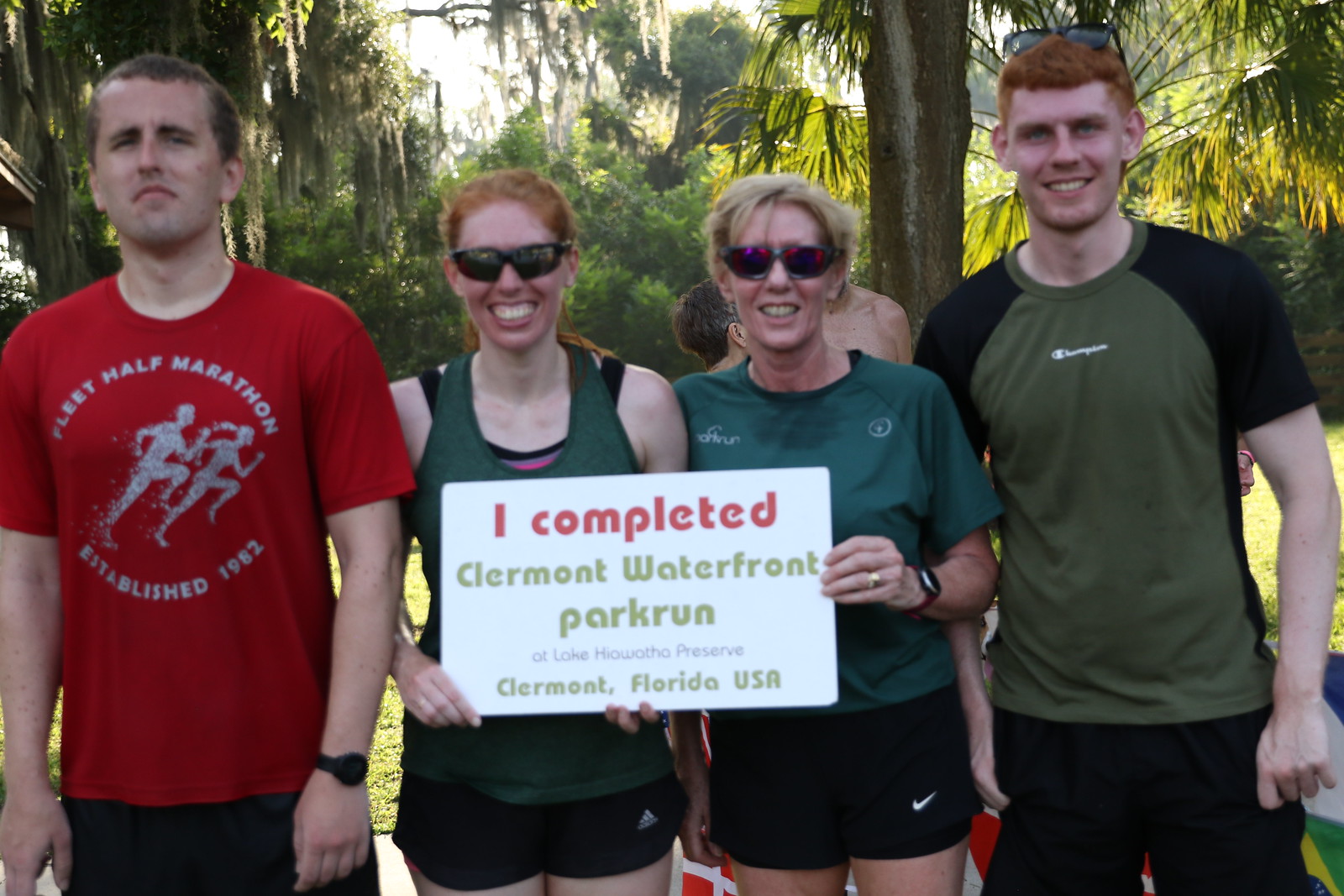This outdoor photograph captures the triumphant moment after a fundraising run at Claremont Waterfront Park in Claremont, Florida, USA. In the image, four individuals are standing amidst a picturesque backdrop of trees, some resembling willows with their long hanging green leaves. The group includes two men and two women, all dressed in runner's attire.

On the left stands a man in a red t-shirt featuring the "Fleet Half Marathon" logo, wearing a watch on his left wrist. Adjacent to him are two women in the center, both sporting green tops, black shorts, and sunglasses, their smiles radiating joy and achievement. They are proudly holding up a white sign that reads, in red at the top, "I completed," followed by, in light green, "Claremont Waterfront Park Run," with "Claremont, Florida, USA" at the very bottom.

To the right, another man with red hair is seen with sunglasses perched atop his head, wearing a green and black shirt along with black shorts. The two men, notably taller than the women, frame the group, adding to the sense of camaraderie and celebration. Behind them, several other runners can be faintly seen, hinting at the larger community event.